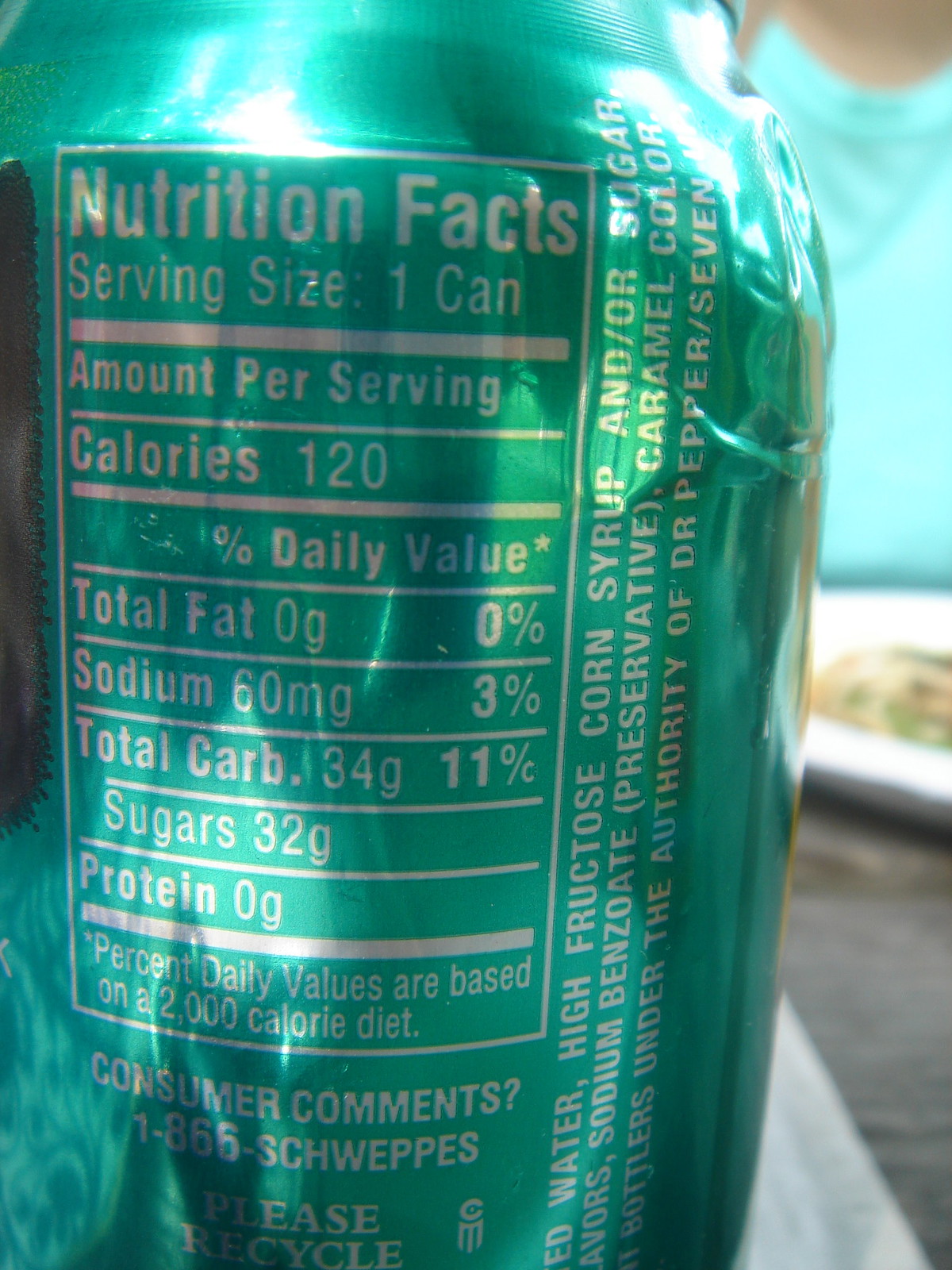In this detailed photograph, the focus is predominantly on a crumpled soda can, capturing the texture and form with its shiny green exterior. The silver text adorning the can stands out clearly against the vibrant green background. To the left side of the can, a rectangular section lists the nutrition facts comprehensively. At the bottom of the can, a phone number for customer comments is visible, reading 1-866-SHWEPS, which suggests the can contains ginger ale, likely from the Schweppes brand. On the right side of the can, a list of ingredients is partially visible. The background is artistically blurred, hinting at the presence of a light teal shirt worn by a person and a possible plate of food, giving the scene a contextual depth that contrasts with the sharp details of the soda can in the foreground.